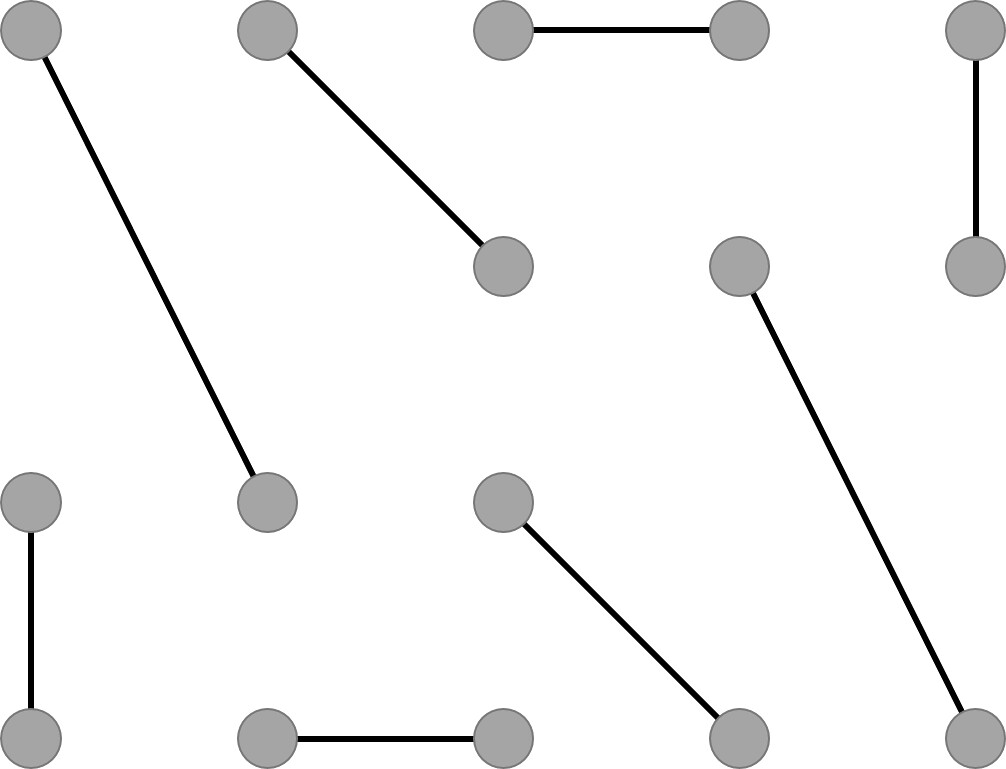The image depicts a complex arrangement of 14 perfectly circular gray points, interconnected by 7 black segments of varying lengths and orientations. Starting from the bottom left corner, there is a small vertical segment, with a small horizontal segment positioned just to the right of it. Above this horizontal segment, a medium diagonal segment extends from the bottom to the top right. Directly above this setup, a larger diagonal segment stretches in a similar direction, intersecting the smaller segment below it.

Further inspection reveals additional segments: another pair of small segments, arranged like a frame, occupies the top right corner. The segments exhibit diverse orientations, including vertical, horizontal, and diagonal alignments, contributing to a visually intricate and symmetrical pattern. The overall geometry forms an intriguing network of connections, showcasing the symmetry and precise placement of each point and segment.